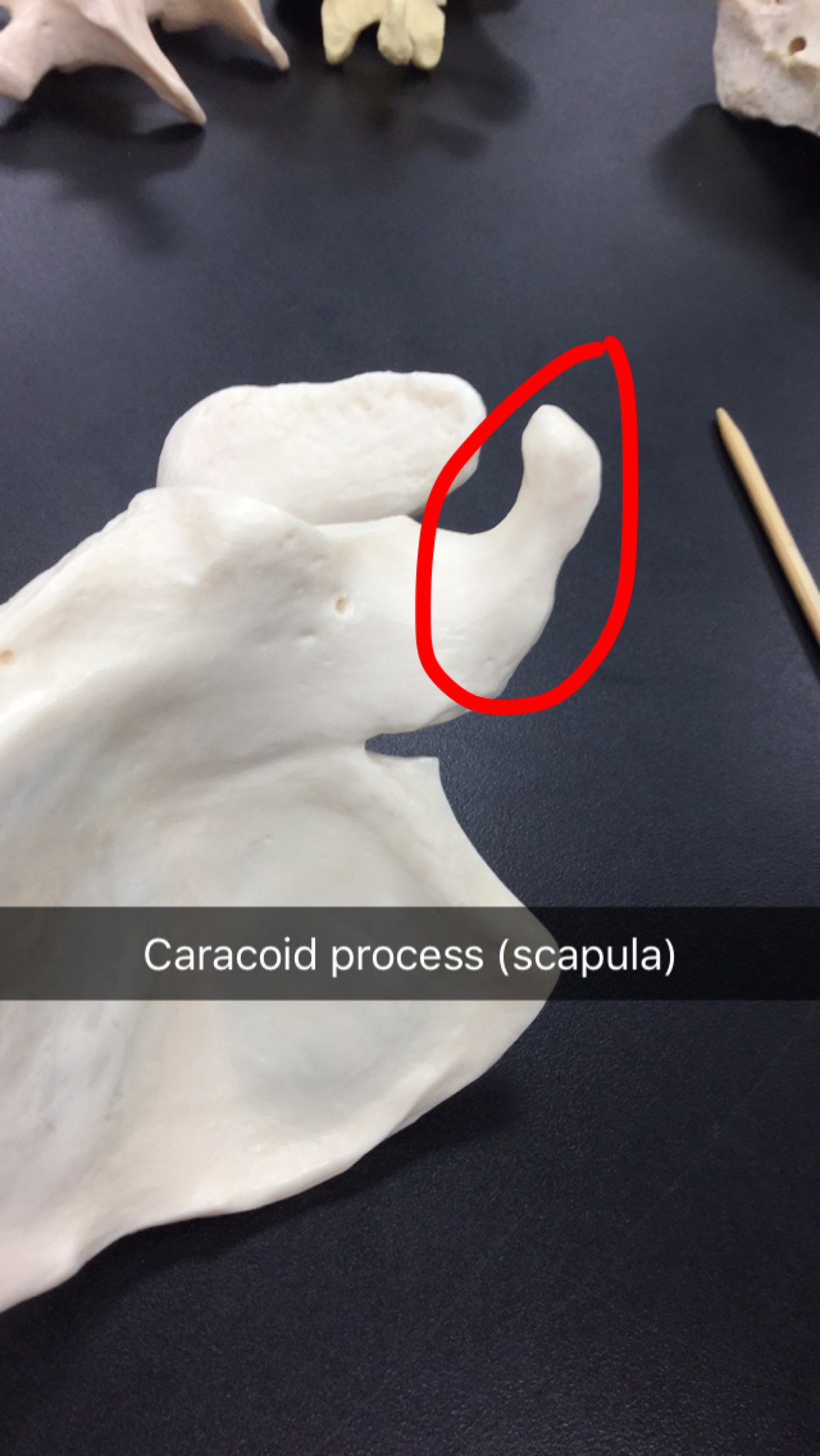The photograph showcases a meticulously bleached white scapula bone centered prominently on a black table. The main feature, labeled "caracoid process (scapula)" in white lettering on a black bar, highlights the primary focus of the image. A portion of the bone is digitally circled in red for emphasis. Adjacent to the scapula is a small wooden probe, and scattered in the background are fragments of other bones, partially visible and slightly darker in color, suggesting age or staining. Overall, the scapula appears smooth with a few pits, and its pristine condition suggests it has been cleaned and polished meticulously.